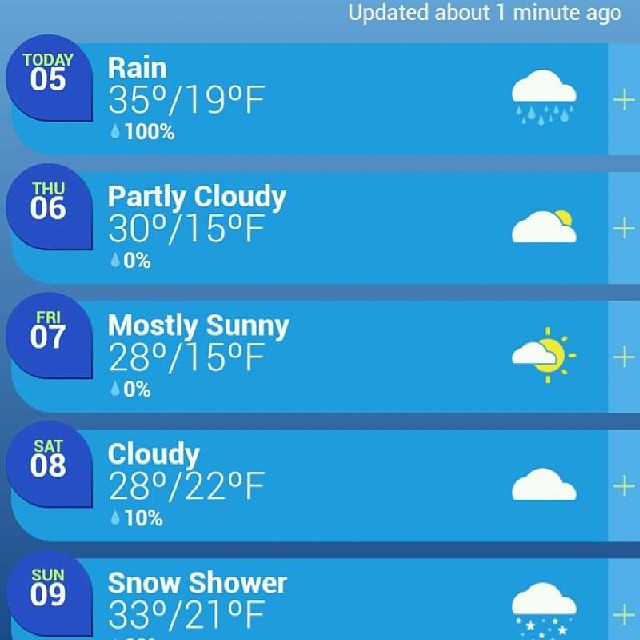The image is a screenshot from a weather forecast application, displaying a five-day forecast. The background of the application is a grayish-blue hue, while each day's forecast is presented in a separate container with a light blue background. In the top right corner of the image, white text reads "updated about one minute ago," indicating the recency of the information.

Each day is organized into rows with a dark blue badge on the left, showing the date and day of the week. The first row, labeled "Today, 05," forecasts rain with a high of 35 degrees and a low of 19 degrees Fahrenheit, and a 100% chance of precipitation. The icon on the far right is a white cloud with blue raindrops beneath it.

The second row, "Thursday, 06," describes partly cloudy weather, with temperatures at 30 degrees high and 15 degrees Fahrenheit low, and a 0% chance of rain. The corresponding icon shows a white cloud with a yellow sun half visible behind it.

The third row, "Friday, 07," indicates mostly sunny conditions with a high of 28 degrees and a low of 15 degrees Fahrenheit, and a 0% chance of rain. The icon here features a smaller cloud with a large sun behind it.

The fourth row, "Saturday, 08," notes cloudy weather, with temperatures of 28 degrees for the high and 22 degrees Fahrenheit for the low, and a 10% chance of rain. The icon is a simple white cloud.

The fifth and final row, "Sunday, 09," forecasts a snow shower, with temperatures of 33 degrees high and 21 degrees Fahrenheit low. The associated icon shows a white cloud with white stars of varying sizes below it.

Each container also includes a small, dark blue badge in the upper corner with a white plus sign in a light blue box, contributing to the compact and organized layout of the forecast information.